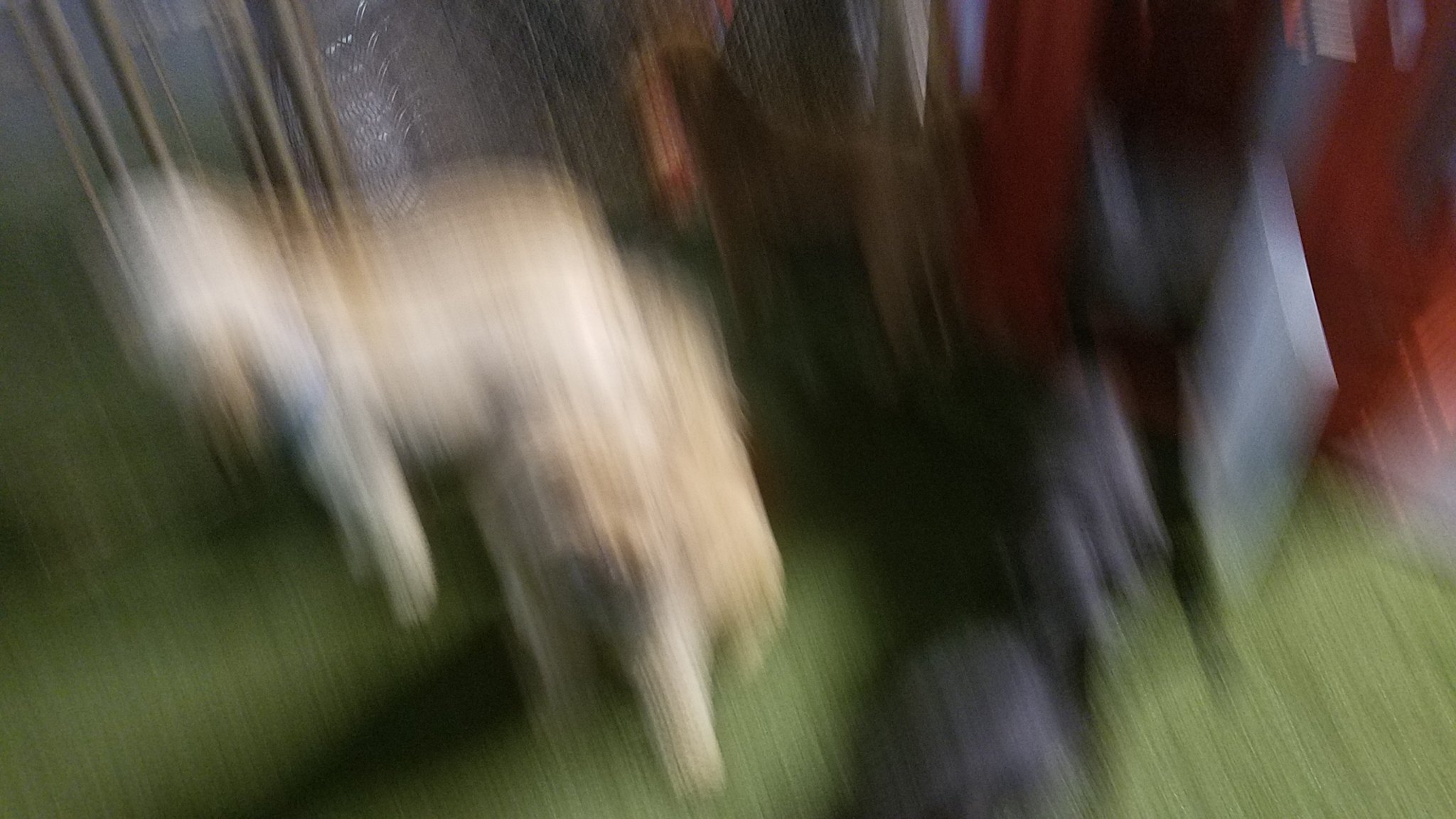This highly blurred color photograph presents a challenging image to decipher. On the left side, there is what appears to be the outline of a dog with pale fur, transitioning to a slightly browner hue around its back. The dog's orientation is ambiguous. To its right, a person dressed in a greyish suit or outfit is partially visible. In front of the person, there seems to be a red object, possibly a bag, though it is difficult to definitively identify due to the blurriness. Surrounding this scene is a greyish metal wall, marked by several narrow, darker grey poles protruding through it. Additional reddish objects are scattered towards the top right and the middle of the composition. The ground at the bottom is covered in green grass, with a notable shadow cast in the middle, seemingly emanating from the dog.